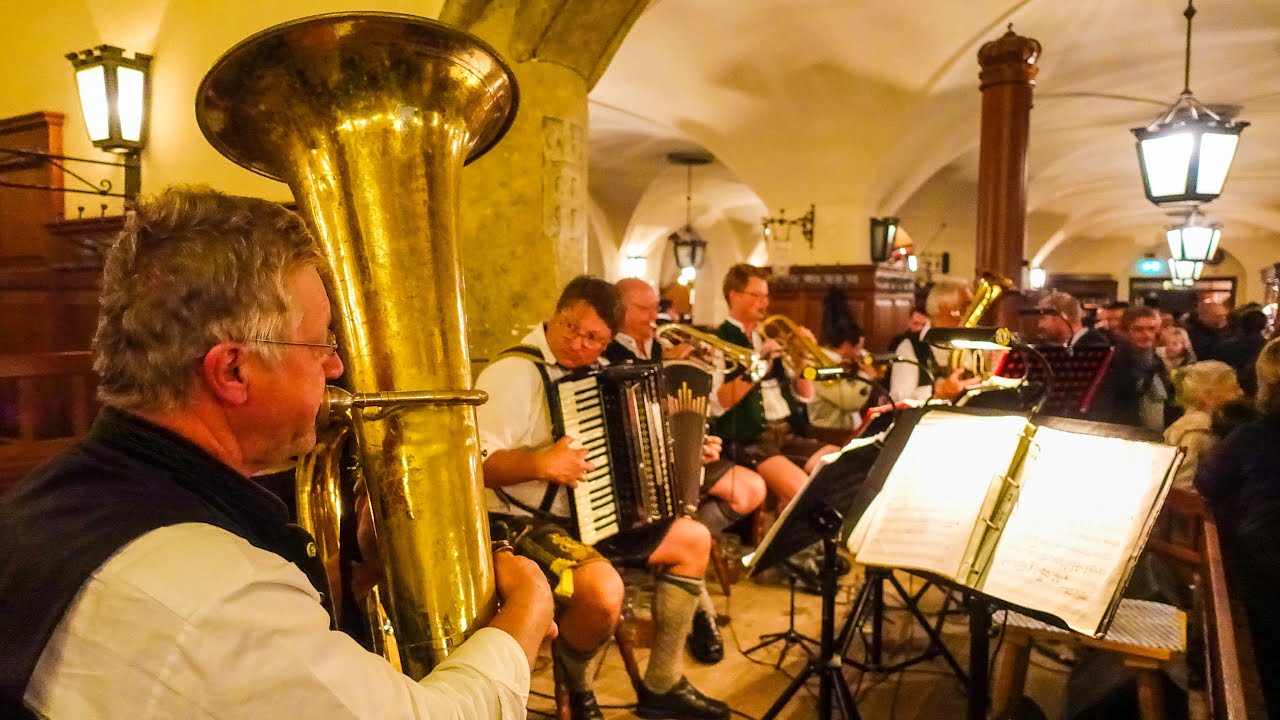The photograph captures an indoor musical event inside a low-ceiling, arched building adorned with hanging lanterns and sconces. The main focal point is an older gentleman of Caucasian descent, seated on the left foreground. He is playing a small tuba and is dressed in a white long-sleeve shirt, a vest, and glasses. The band consists of several older white men, most of whom are wearing vests and lederhosen with knee-high socks, and they are playing an array of brass instruments including trumpets and possibly a French horn, while one plays an accordion and another a piano. The men are seated behind black music stands with music sheets. On the right side of the image, there is a blurred view of the audience seated at tables, enjoying the performance. The room’s ceiling features cream-colored plaster with wooden pillars extending down, creating a cozy and quaint atmosphere.